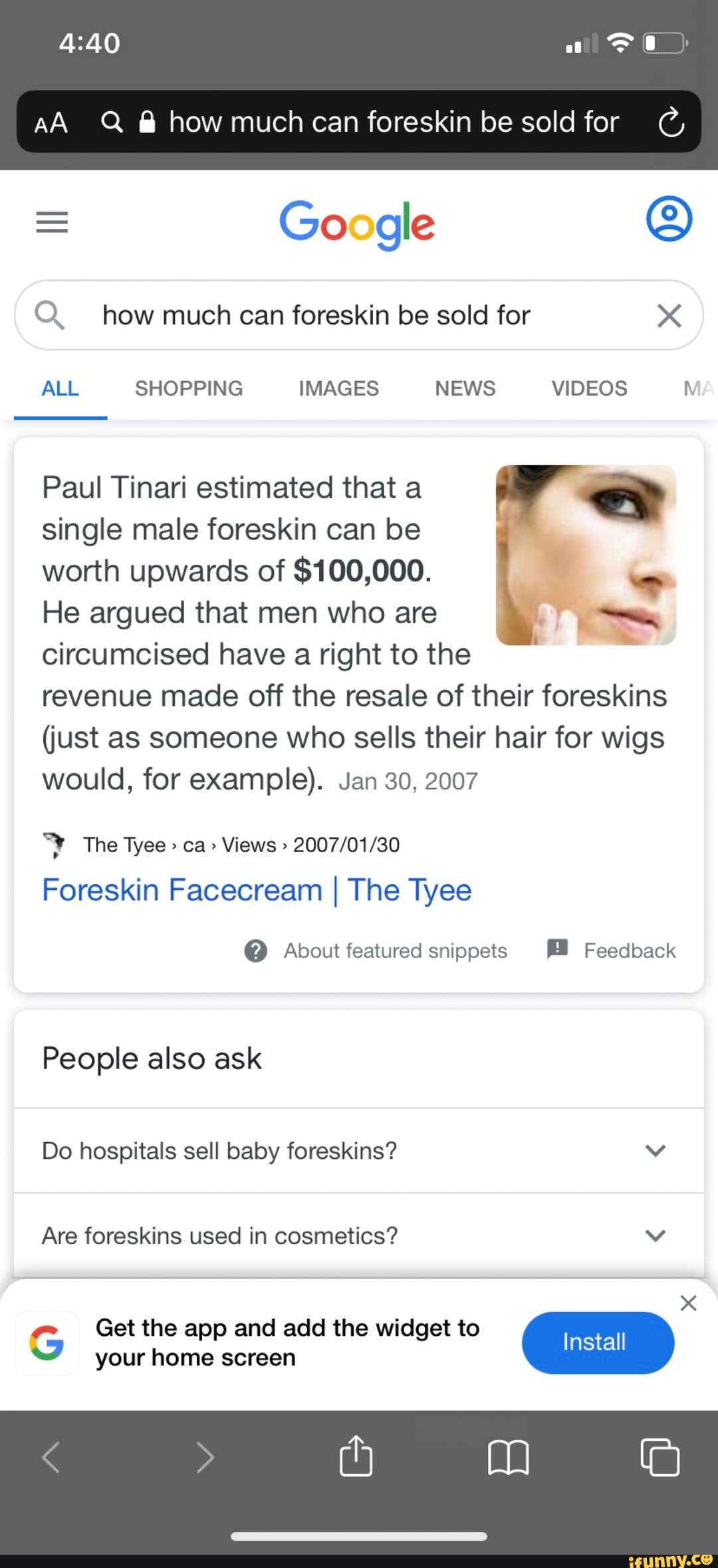The image depicts a Google search result page displayed on a user's cell phone home screen. The screen features a dark gray banner at the top, showing the time "4:40" in white text on the left-hand side. To the right, there are two signal bars and a battery icon at approximately 20%. Directly below this banner is a black search bar containing the query in white text: "how much can foreskin be sold for?"

Below the search bar, the Google result page appears on a white background. Centered at the top is the Google logo in its signature colors. To the left of the logo are three horizontal bars, and to the right is a bright blue icon depicting a person. Beneath this setup is another search bar, this one with black text repeating the query: "how much can foreskin be sold for?"

The prominent search result includes a piece of text accompanied by an image. The image shows an androgynous individual with short hair, who is touching their jawline with two fingers, seemingly highlighting their smooth skin. The text reads: "Paul Tenari estimated that a single male foreskin can be worth upwards of $100,000. He argued that men who are circumcised have a right to the revenue made off the resale of their foreskins (just as someone who sells their hair for wigs would, for example)." Below this, in bright blue text, the words "foreskin face cream" and "The Tyee" (T-Y-E-E) are highlighted, indicating a possible source or related article.